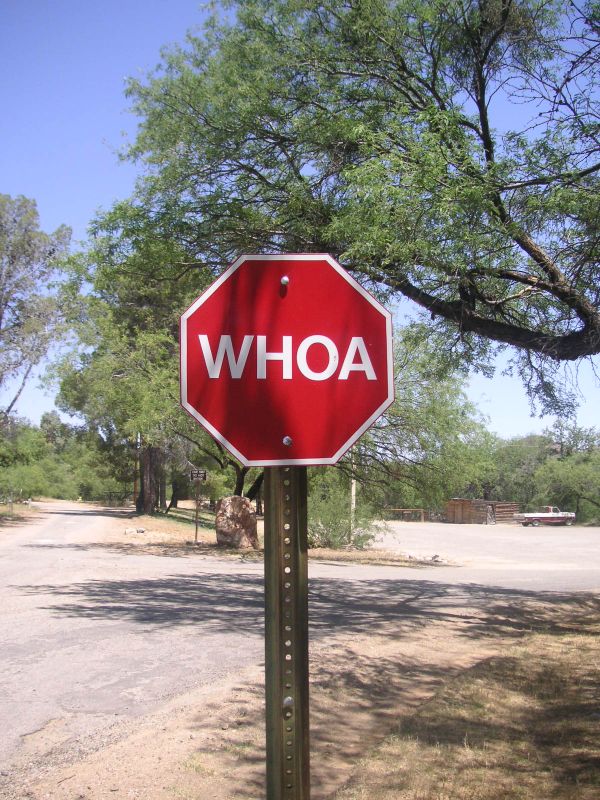This photograph captures a unique and unusual street sign set against a rustic country backdrop. The sign, shaped like a standard red octagon with a white border, is prominently fixed atop a short metal pole marked by numerous small round holes. Unlike typical stop signs, this one boldly displays the word "WHOA" in all-cap white letters at its center. The sign is secured with screws visible at its top and bottom. Behind the sign, a dirt road stretches out, flanked by trees with branches reaching up, casting a natural, earthy ambience. In the background, a light blue sky fades to nearly white near the horizon, adding a serene touch to the scene. To the right, there's a gravel parking area where an old brown and white pickup truck is parked, its front end facing right. A large rock also sits in this area, adding to the rural charm of the setting. Scattered dry grass and patches of green trees provide a vivid natural setting, enhancing the overall rustic feel of the image.